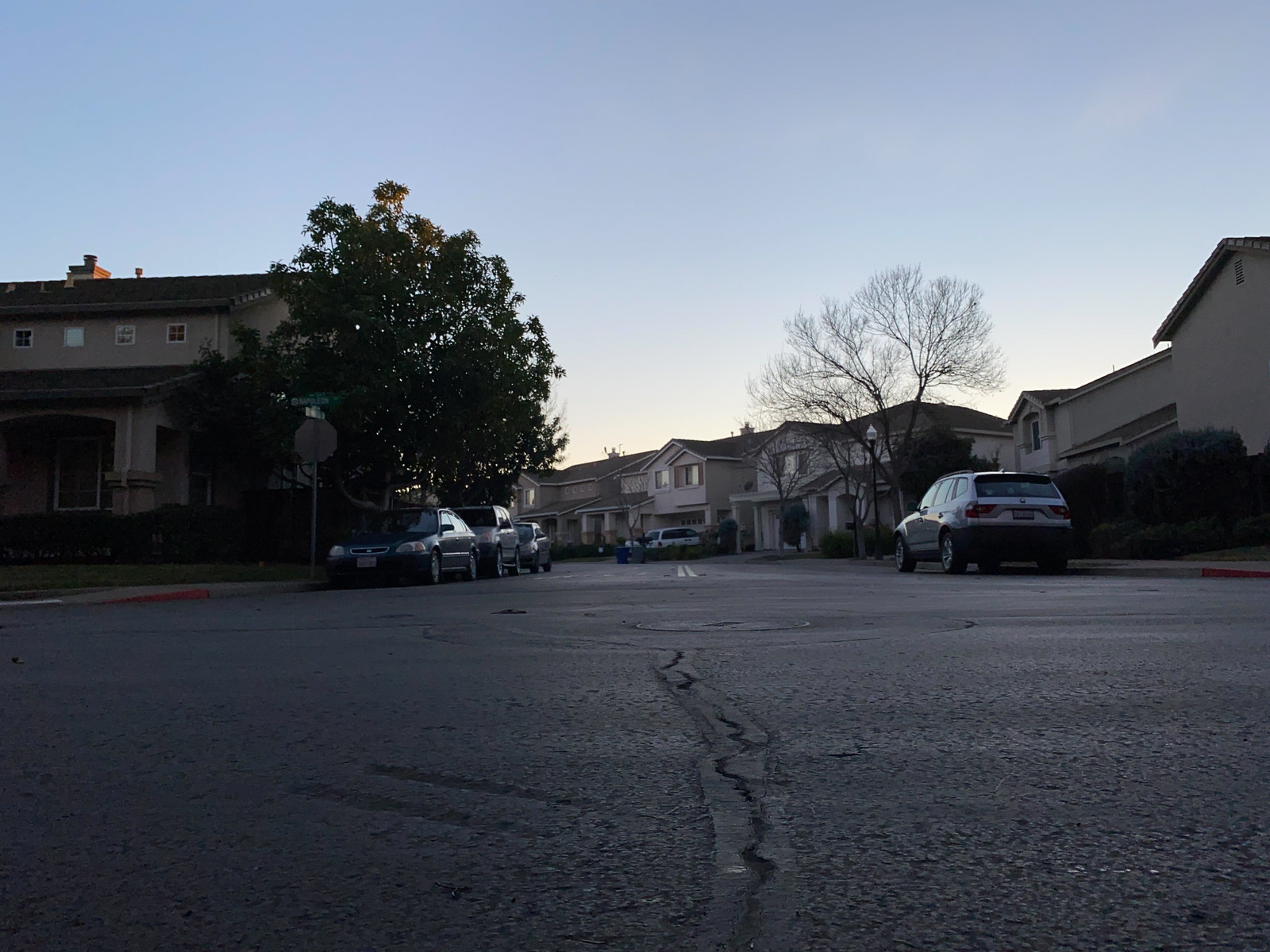This striking ground-level photograph captures a tranquil residential street. The asphalt pavement in the foreground is marked with visible cracks, providing a rustic texture to the scene. Dominating the visual center is a stop sign seen from the rear, paired with two green street signs—one facing the viewer and the other pointed away.

Parked along the curb, a dark-colored Honda Civic and a silver BMW SUV lend a suburban authenticity to the composition. The background features two-story homes adorned with stucco exteriors in neutral shades of white and gray. Each house sports a hip-shaped roof, adding architectural interest to the neighborhood.

Flanking the street, two trees present a stark contrast: a lush, verdant tree on the left and a barren one on the right. A tall streetlight with a black pole and a white thatched top further punctuates the scene. In the distance, curbside trash bins—a blue one and a gray one—sit dutifully in front of a house, hinting at the everyday rhythm of life in this serene enclave.